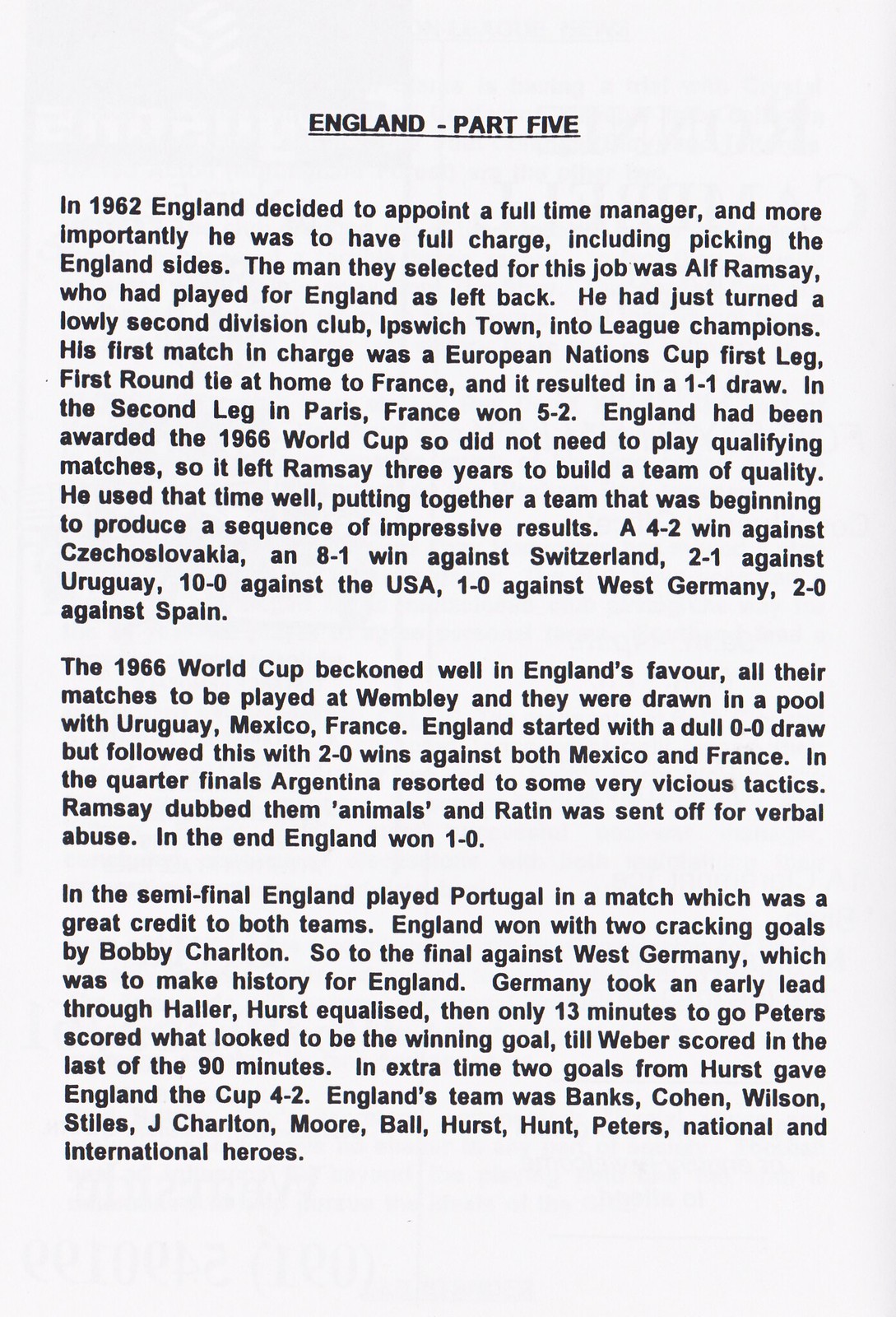The image is a black and white photograph of what appears to be an article. The article is presented on a plain, white sheet of paper, likely a standard 9 1⁄2 by 11 inches, with all text in black, resembling a typewriter font. At the top center of the page, the heading reads "England Part 5." The text recounts significant events in English football history starting in 1962 when England decided to appoint a full-time manager with complete control over team selection. The chosen manager was Alf Ramsey, a former England left-back who had recently led the second division club Ipswich Town to become league champions.

The narrative details Ramsey's tenure, beginning with his first match in charge in the European Nations Cup, which led to a 1-1 draw at home against France and a subsequent 5-2 victory in Paris. With England set to host the 1966 World Cup and thus not needing to play qualifying matches, Ramsey had three years to build a formidable team. During this period, England achieved impressive results, including victories over Czechoslovakia (4-2), Switzerland (8-1), Uruguay (2-1), the USA (10-0), West Germany (1-0), and Spain (2-0).

The article continues by covering England's journey through the 1966 World Cup. In the group stage, England started with a 0-0 draw against Uruguay but secured 2-0 wins against both Mexico and France. The quarterfinal against Argentina was contentious, marred by rough play, leading Ramsey to call the Argentine players "animals"; England won the match 1-0. In the semifinal, Bobby Charlton's two goals secured a victory against Portugal. The climax of the account is the final against West Germany, where Geoff Hurst's hat-trick and Martin Peters' goal led England to a historic 4-2 win in extra time, clinching the World Cup. The final whistle saw England's team — consisting of Banks, Cohen, Wilson, Stiles, J. Charlton, Moore, Ball, Hurst, Hunt, and Peters — celebrated as national and international heroes. The entire text is in black on the solid white background.